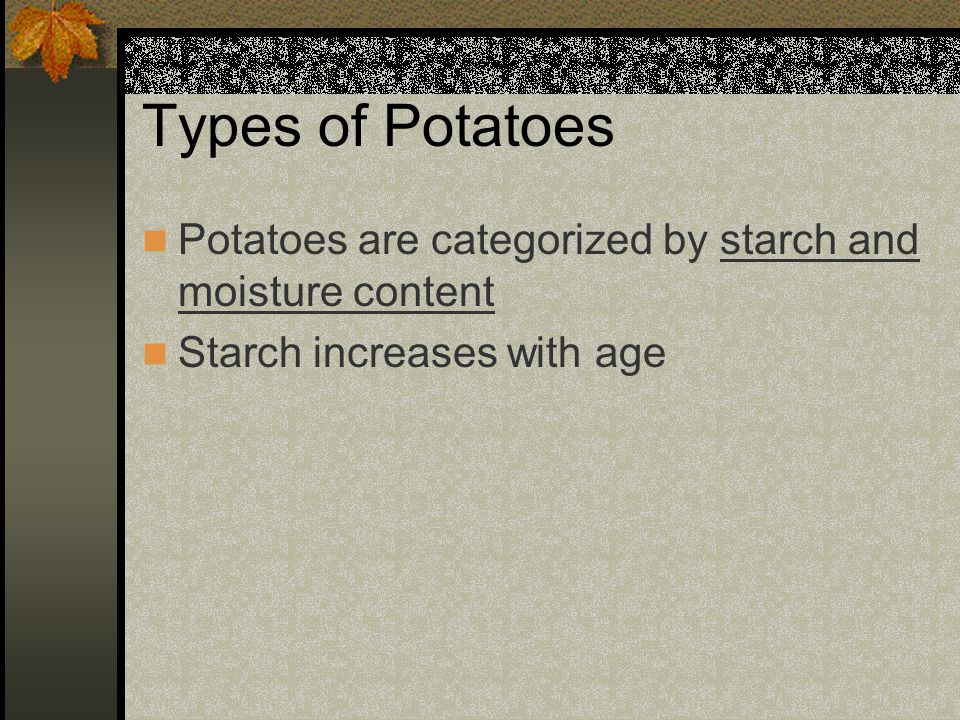This image features a PowerPoint slide titled "Types of Potatoes" in black Arial font. The background is primarily olive green with a dark brownish-beige border at the top. In the top left corner, there is an orange leaf graphic that gives an autumn feel. Below the title, there's a decorative textured black and white strip. The slide contains two bullet points, marked by orange square bullets. The first bullet point states, "Potatoes are categorized by starch and moisture content," with the words "starch and moisture content" underlined. The second bullet point notes, "Starch increases with age." There is a vertical thick dark gray stripe running along the left side of the slide, enhancing its visual structure.